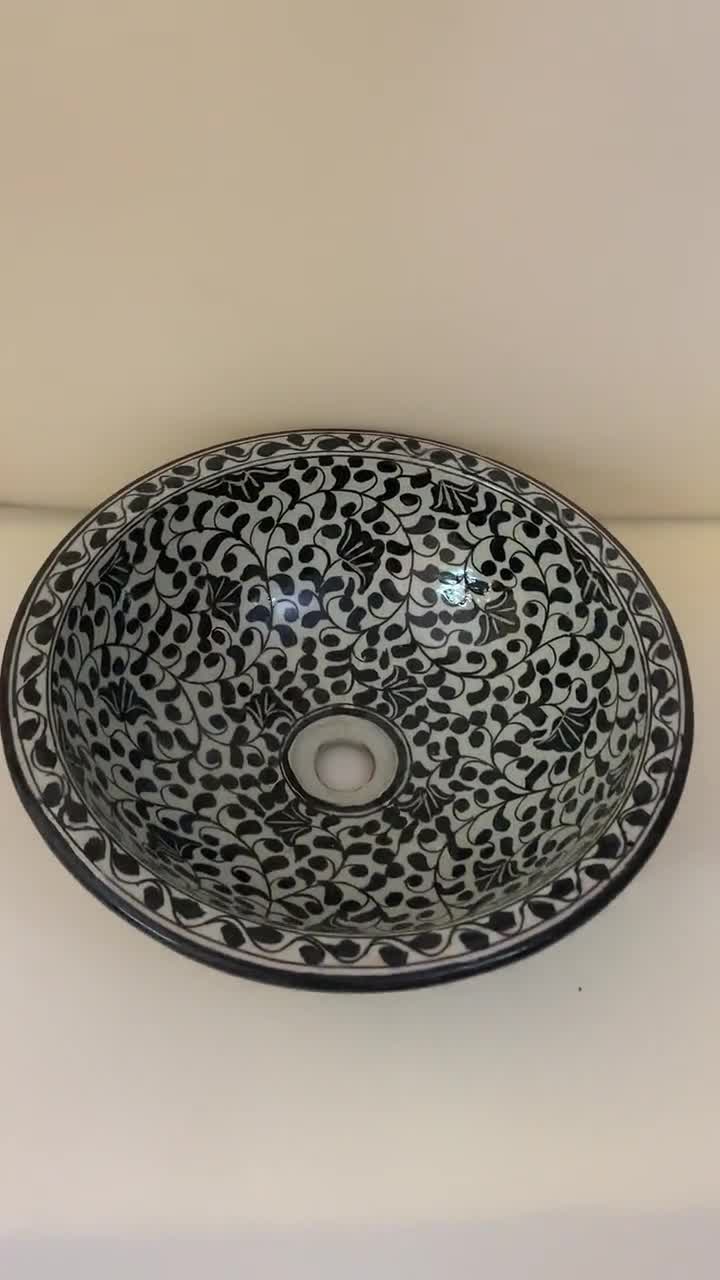A strikingly decorative and ornate bathroom sink commands the forefront of the image, nestled securely on a smooth, cream-colored surface that harmonizes with the cream-toned background wall. The sink itself stands out as a stunning centerpiece, designed in a graceful, round, bowl-like shape. 

Intricate and elegant black vines meander along the rim, adorned with delicate black leaves, adding a touch of sophisticated artistry. These vines artistically weave their way into the bowl of the sink, flourishing into a more elaborate pattern that includes black leaves and blossoms, all set against a pristine white background. The detailed botanical design exudes a timeless charm and a serene natural beauty. 

At the heart of this beautifully crafted sink lies a substantial cut-out circle, presumably for drainage, seamlessly incorporated into the artistic design, reflecting both functionality and aesthetic appeal.